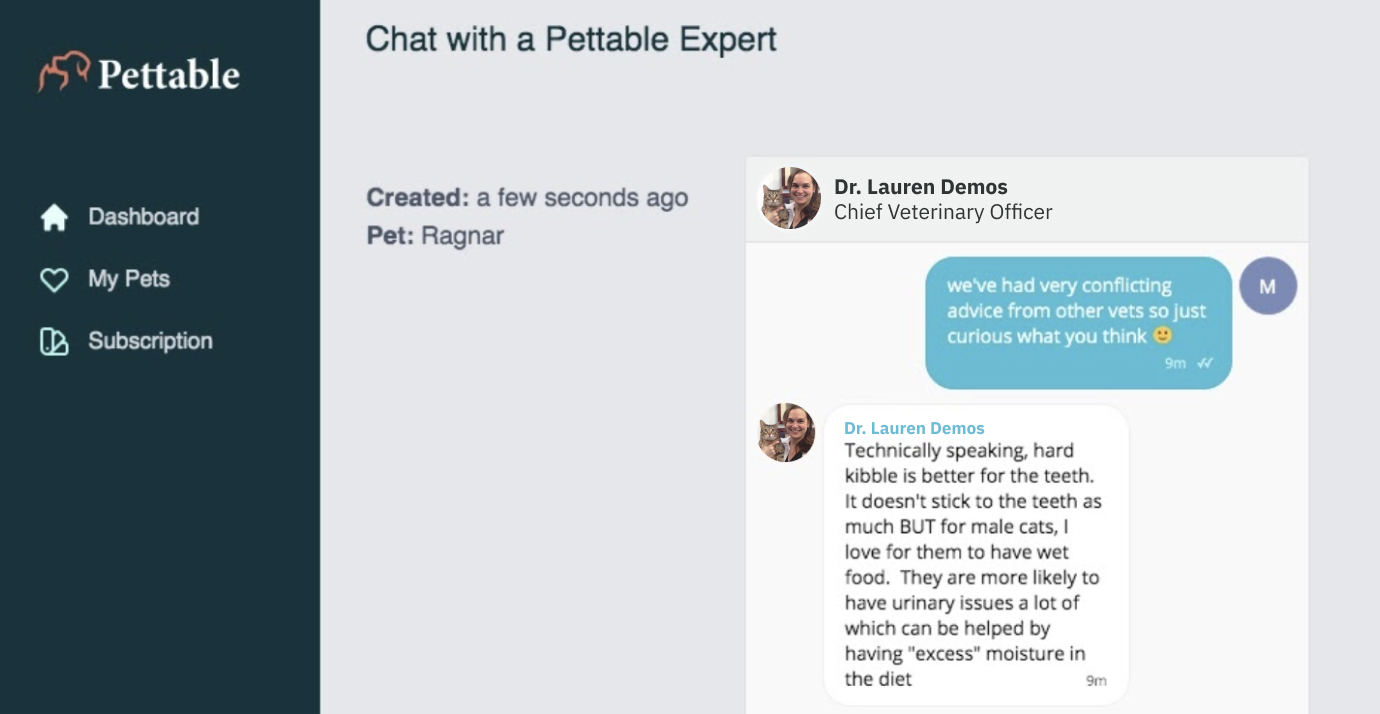On the left side of the image, there is a grayish dark blue background featuring the word "Pedible" in a bold, white Times New Roman font at the top. Below this text, the silhouettes of a cat and a dog are shown, with the cat nuzzled into the dog's neck. This silhouette is framed by an orange border. Beneath this area, there are three menu options: 

1. "Dashboard" with a white house icon — this option appears to be selected as it is bolder compared to the others.
2. "My Pets" with a white heart icon.
3. "Subscription" with an icon of three cascading phones.

To the right, the background shifts to light gray. At the top left of this section, it says "Chat with a Pedible Expert" in black text. Underneath that, "Created: a few seconds ago" is noted, with "Created:" in bold gray lettering. Below that, "Pet: Ragnar" is listed, with "Pet:" in bold.

Moving further to the right, a conversation is shown. The user is interacting with Dr. Lauren Demos, who is identified as the Chief Veterinary Officer. Her profile icon, which shows her with long light brown hair and her cat, is displayed in a circle to the left. The user's message reads: "We've had very conflicting advice from other vets so just curious what you think 🙂." Below, Dr. Lauren Demos responds: "Technically speaking, hard kibble is better for the teeth as it doesn’t stick to the teeth as much. But, for male cats, I LOVE for them to have wet food. They are more likely to have urinary issues, which can be helped by having excess moisture in the diet."

This detailed caption provides a clear and comprehensive description of the image, ensuring all elements are articulated accurately.